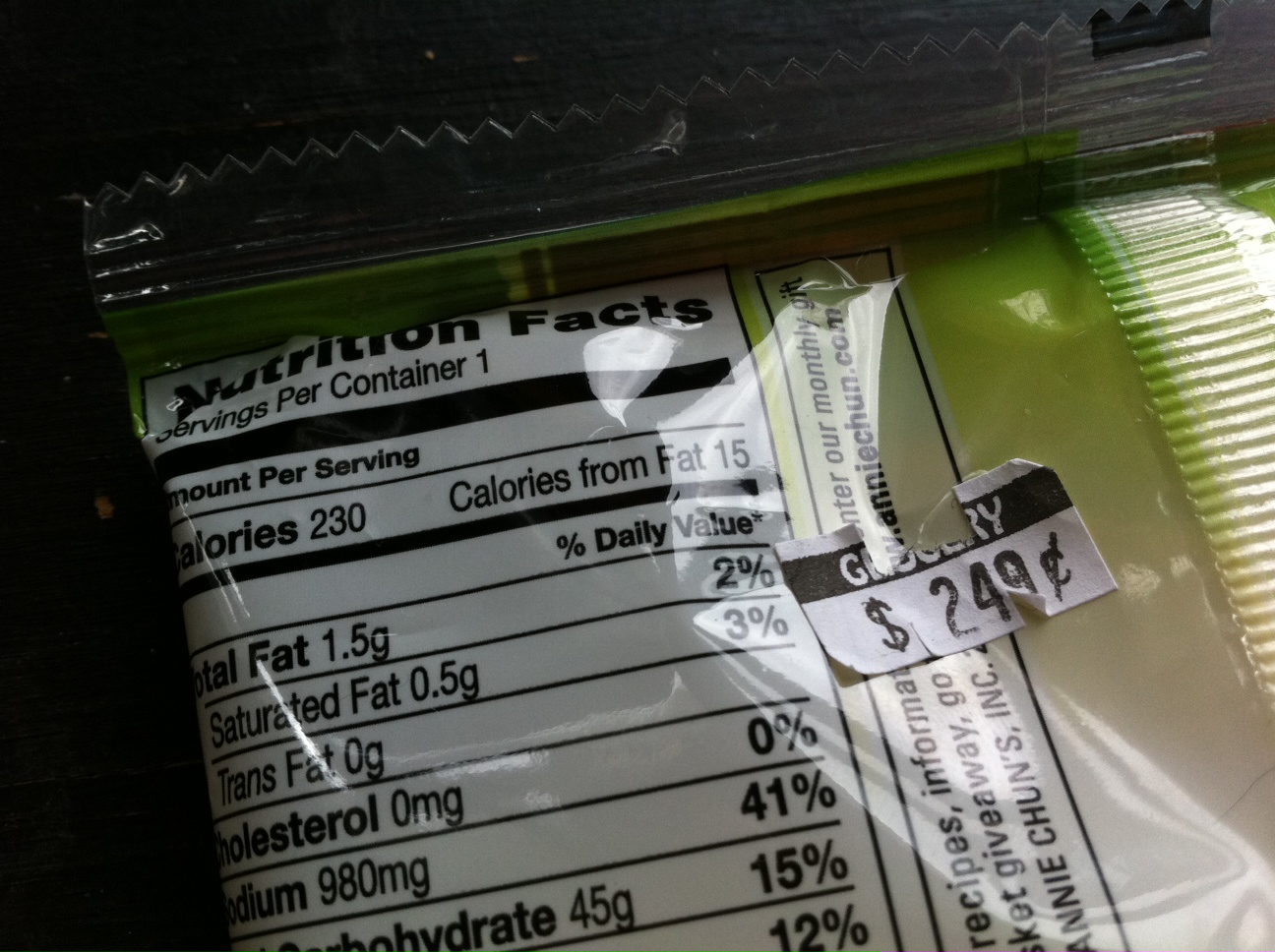The image depicts the back of a plastic food package, likely a snack such as chips or candy, taken from a horizontal perspective. Primarily, the nutrition facts are visible and indicate the following details: servings per container are 1, with 230 calories, 15 calories from fat, 1.5 grams of total fat, 0.5 grams of saturated fat, 0 grams of trans fat, 0 milligrams of cholesterol, 980 milligrams of sodium, and 45 grams of carbohydrates. The package itself features a shiny, dark green material that transitions into lighter shades of green, especially towards the seal, which is black. Additionally, there is a partially torn white and black price sticker indicating $2.49, with fragments of the word "grocery" on it. The bag has a reflective quality, giving off light from the right side, and part of an ingredient list is visible, but not fully readable.